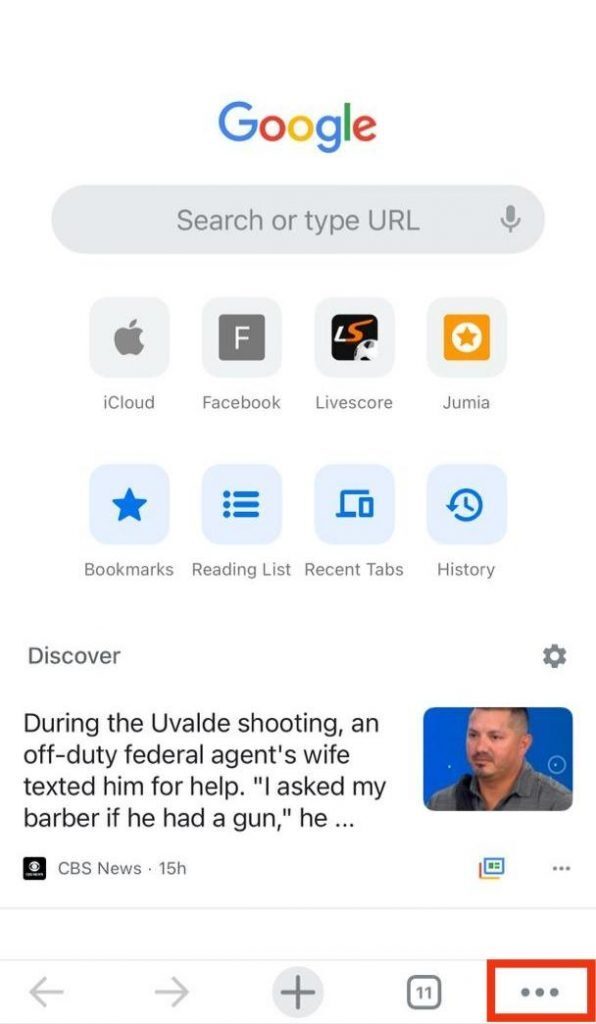This image depicts a browser tab with various details. At the top, the Google logo is prominently displayed in its recognizable blue, red, yellow, and green colors. Below the logo is a URL search bar featuring a gray microphone icon. Several saved bookmarks are visible, including an "iCloud" tab with a gray Apple logo, a "Facebook" tab with an "F" logo, a "Live Score" bookmark indicated by an "LS" logo and a soccer ball, and a "Jumei" tab with an orange star logo at the center. 

To the right, there is a bookmarks section marked by a blue star, a reading list symbolized by various dots and lines on a blue background, a recent tabs section denoted by icons of a computer and a smartphone, and a history button illustrated by a circular clock with a backward-facing arrow. A discovery section is also present, marked by a gear icon.

The headline of the page reads, "During the Uvalde shooting, an Occuty federal agent's wife texted him for help. I asked my barber if he had a gun." This news article is from CBS News and was posted 15 hours ago. Beneath the headline, there is an image of a man in a button-down shirt. At the bottom of the browser, a series of buttons are visible: a backward arrow, a forward arrow, a gray plus sign, a tab icon displaying the number 11, and three gray dots outlined in red.